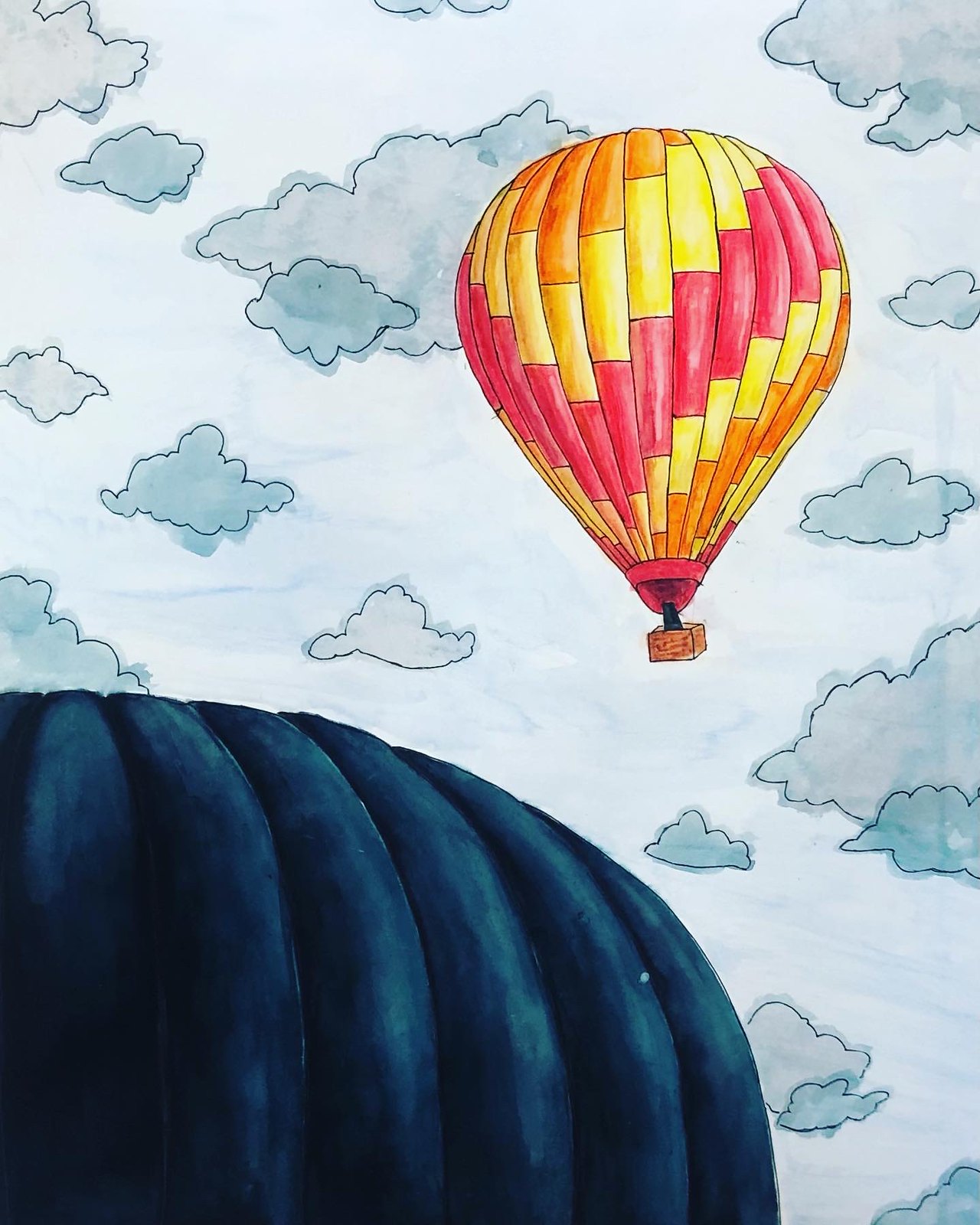The artwork before me features two hot air balloons soaring majestically against a vibrant sky. The balloon in the foreground boasts a vibrant palette, with sections of orange, yellow, and pink, creating a striking contrast with the serene sky. Beneath this colorful canopy, the basket is clearly visible, suggesting a space for passengers to enjoy their aerial journey. In the bottom left corner, the outline of a second hot air balloon is discernible, its upper section adorned in shades of blue. The remainder of this balloon fades out of view, adding a sense of depth to the composition. The background is a panoramic display of blue skies interspersed with clouds, rendered in varying hues of blue and grey, showcasing intricate details that enhance the overall realism of the scene.